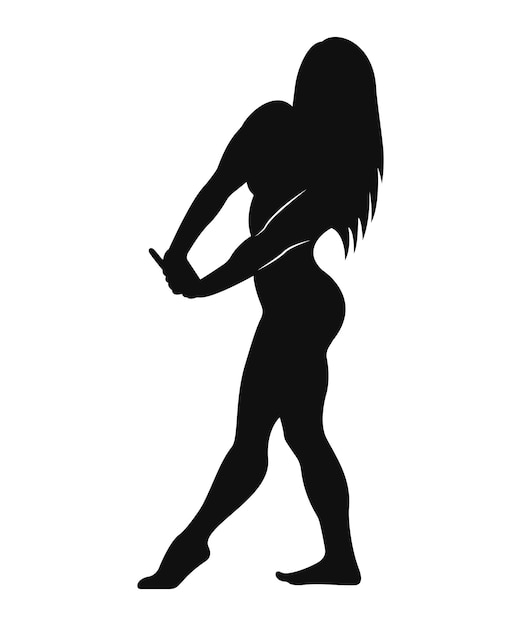The image depicts a simple, yet striking black silhouette of a poised, strong female figure against a solid white background. She is facing left with her arms extended and clasped in front of her, reminiscent of a stretching motion one might use to crack their knuckles. Her right leg is prominently extended forward, almost hyper-extended, with the foot raised and pointed in a manner suggestive of wearing high heels. The depiction hints at a muscular build, evoking the stance of a bodybuilder during a pose. Her long hair cascades down, and no facial features are visible. To add definition, there is a distinctive white cutout around her left arm, emphasizing its form and ensuring clarity within the silhouette. Overall, it is a detailed and intentional portrayal that emphasizes strength and grace.